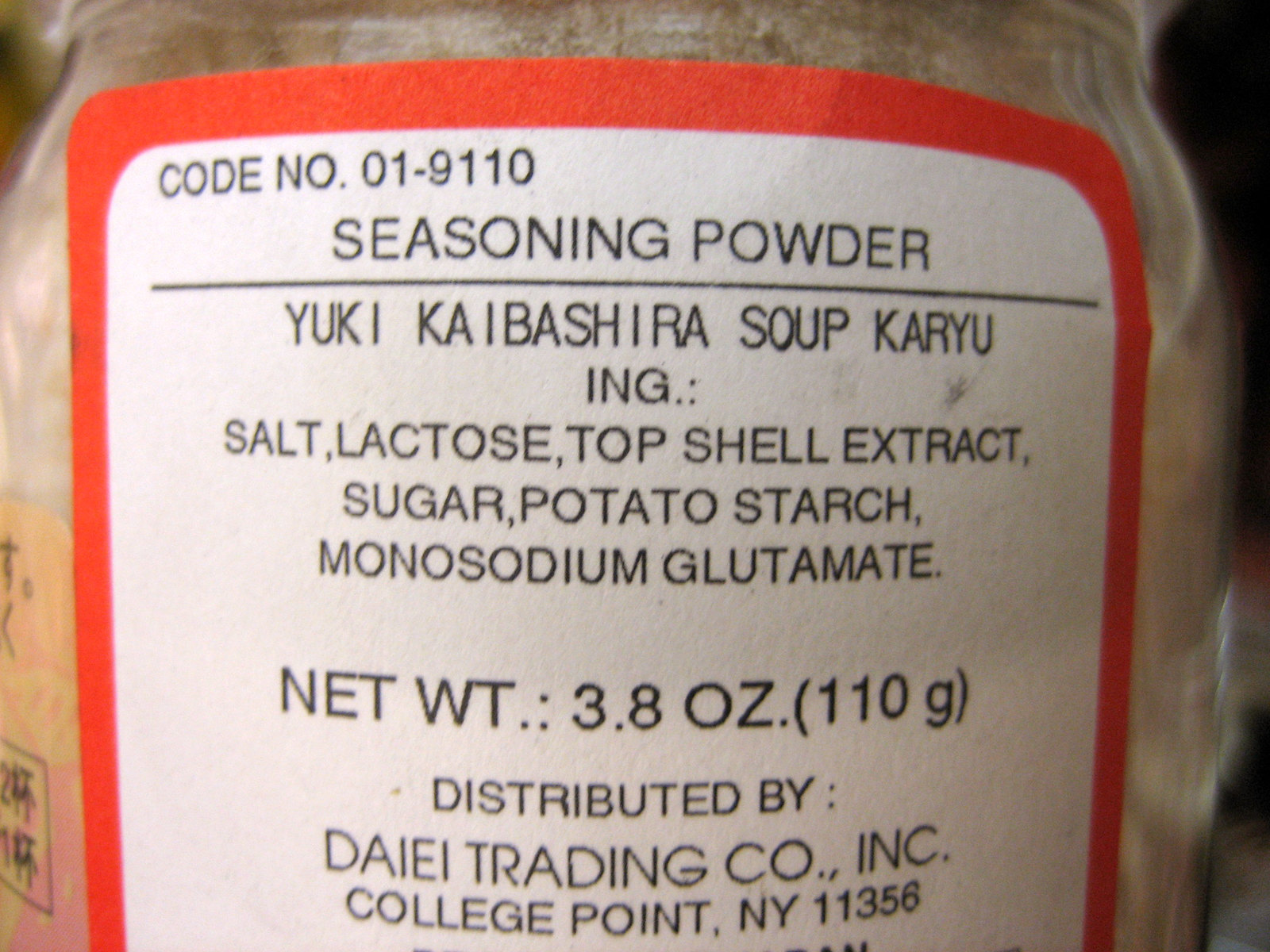The image features a close-up of a labeling on a clear glass jar containing a light tan or orange-y colored seasoning powder. The primary label is a white paper with a noticeable wrinkle, surrounded by a bold red outline, and featuring black printed text. The powder seems to be a seasoning mix that includes ingredients such as salt, lactose, top shell extract, sugar, potato starch, and monosodium glutamate. The label prominently displays many elements in what appears to be Korean or Japanese, mentioning components like yuki, kabasheria, soup, and kairu, hinting it might be intended for soup seasoning. Additionally, a smaller, beige label with black print can be faintly seen on one side of the jar. The product is from Dye Trading Company, College Point, New York. The background is black and the jar is placed on a light-colored surface. Due to the zoomed-in perspective, only the top half of the label is clearly visible, displaying intricate details of its design and content information.